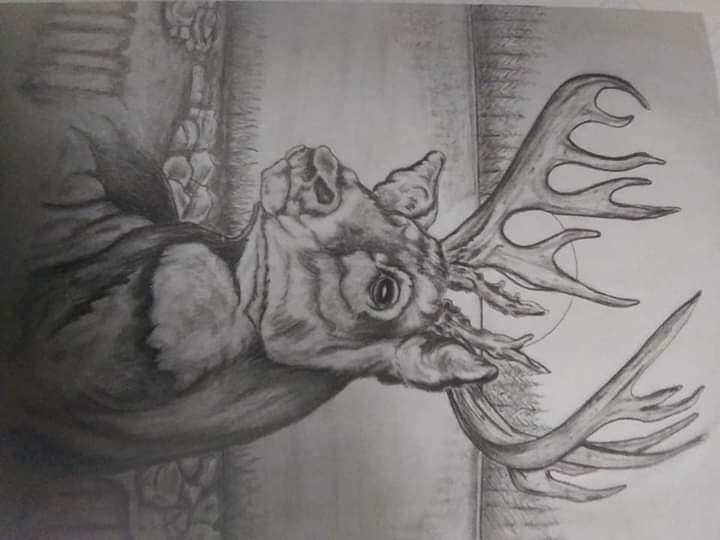The image is a detailed pencil or charcoal drawing of a deer, specifically a buck, featuring its head, neck, and impressive antlers, which appear to have 11 or 12 points. The deer’s face is rendered with a weathered but stoic expression, indicative of age and experience. The background includes a lightly shaded lake with some rocks in the foreground and a cluster of pine trees in the distance. Notably, there is a large half-circle, presumably the rising sun, situated behind the antlers. The drawing is of high quality and appears professionally done. The entire scene is rotated 90 degrees to the right, requiring viewers to adjust their perspective.